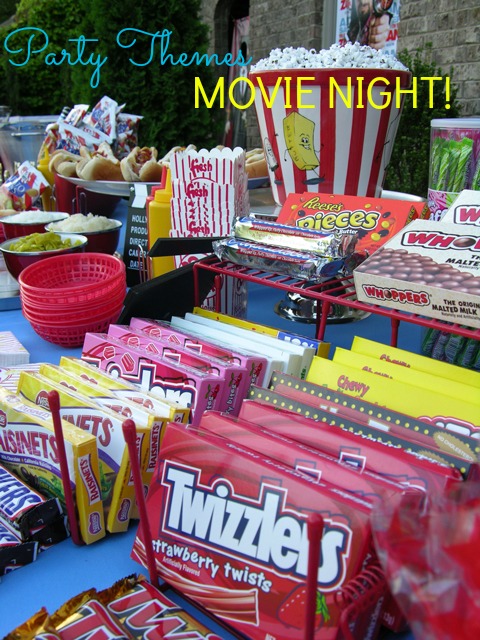This vibrant, portrait-oriented color photograph captures a well-stocked concession stand against a backdrop of a two-colored brick building. The upper left corner features the text "Party Themes" in light blue cursive, while the upper right corner has "MOVIE NIGHT!" in bold, thin yellow all-caps font. The stand is adorned with a variety of snacks displayed on red wire shelving, including prominent front-row packages of Twizzlers, Raisinets, Snickers, Whoppers, Reese's Pieces, and Three Musketeers bars. Above these, a larger red and white striped popcorn container brimming with popcorn is visible, accompanied by smaller popcorn boxes. Additionally, red plastic baskets, a platter of hot dogs, and various condiments like potato salad and relish can be seen in the upper left corner. A blue tablecloth covers the table, enhancing the colorful and appetizing array of movie snacks, perfectly capturing the essence of a festive movie night theme.